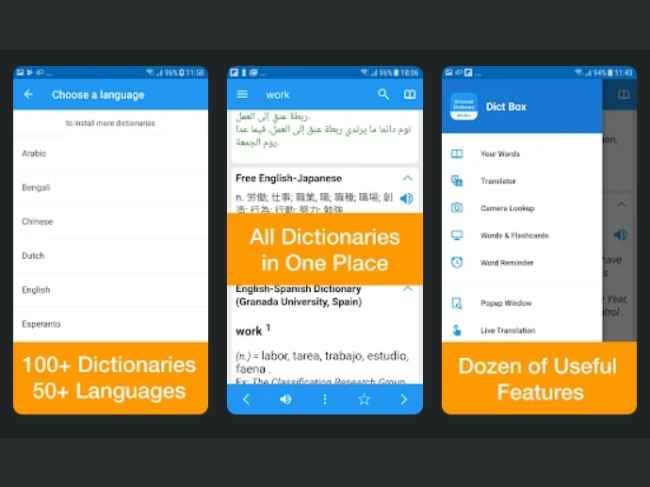The image displays a website with a black background, featuring three identical-sized graphics aligned vertically from left to right. Each graphic resembles a webpage with varying content but shares a similar structure.

The first graphic on the left side has a dark blue banner at the top, displaying icons for battery strength, cell signal, Wi-Fi signal, and the time. Below this, a larger blue banner with white text reads "Choose a Language." Under this section, navigation elements include a left arrow. The language options listed are Arabic, Chinese, Dutch, English, and Esperanto. An orange banner below highlights "100+ Dictionaries, 50+ Languages."

The central graphic contains the same dark blue banner at the top. Below it, bold text reads "Work with a magnifying search" followed by some foreign text. An orange banner states, "Free English to Japanese, All Dictionaries in One Place." At the bottom, a blue banner features icons for a left arrow, microphone, a three-dot vertical menu, a star, and a right arrow.

The third graphic on the right mirrors the same dark blue top banner. It includes a drop-down menu labeled "DICT Box" and a white background section with options such as "Your Words, Translate, Camera Look Up, Words and Flashcards." An orange banner at the bottom mentions "Dozens of Useful Features."

Overall, the graphics seem to illustrate different interfaces or promotion pages for a digital dictionary or translation tool.